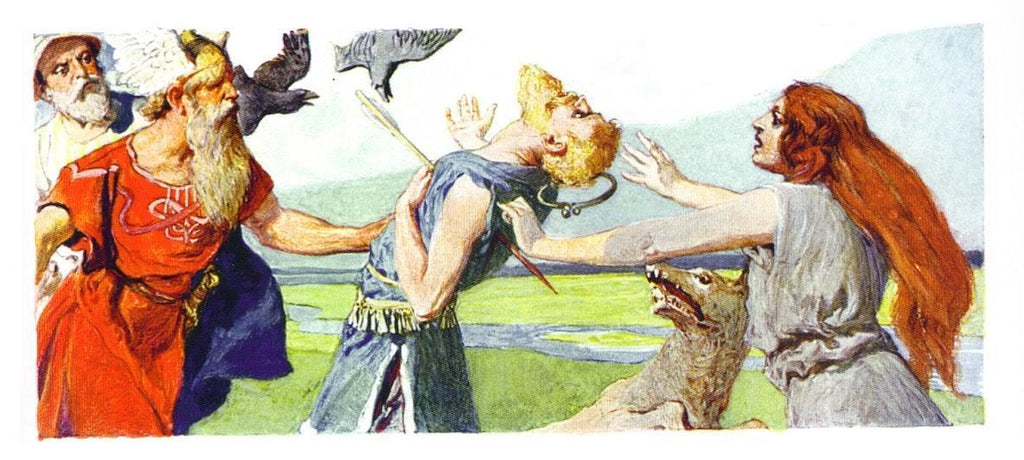This intricate painting captures a dramatic scene full of emotional intensity and symbolism. Positioned prominently on the right, a female figure with flowing orange hair is dressed in a white dress. She extends her arms in a gesture of anguish or plea towards a male figure in a blue robe with golden hair. The male appears to be in deep distress, impaled by a red-stained stick or possibly a knife, suggesting he has been grievously wounded.

To the left, another male figure, distinguished by his white hair and beard, is clad in a red robe. His stance and the presence of the weapon suggest he is the assailant. Behind him stands yet another male figure, also with white hair and beard, dressed in a blue robe. He seems to be restraining or pulling back the red-robed assailant, adding to the chaotic and violent atmosphere.

In the backdrop, two grey birds are visible, adding a further layer of symbolism and depth to the scene. The detailed expressions and positioning of the figures, combined with the dynamic composition, evoke a powerful narrative of conflict, betrayal, and despair.